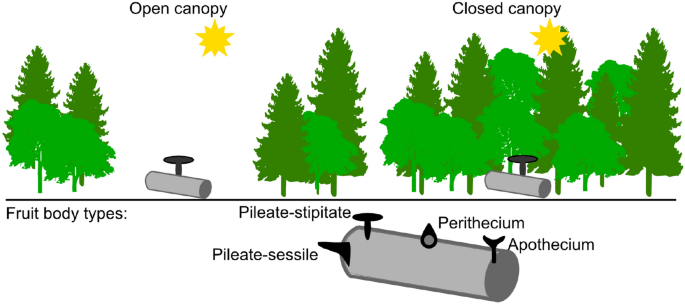This image is a detailed infographic illustrating the types of forest canopies and a related cylindrical tool. On a horizontal timeline, from left to right, it depicts open canopy and closed canopy tree arrangements. The left side, labeled "Open Canopy," features tufted fir and pine trees with dark and light green shades, separated by an open area with a sun depicted above, symbolizing a sparse forest cover. The right side, labeled "Closed Canopy," shows dense groupings of fir and pine trees without any gaps, also with a sun shining above, indicating a thick forest cover. Below the trees, a silver, cylinder-shaped tool with black text labels for its parts is displayed, connected to the concepts of "fruit body types," specifically "pilate" and "stipulate" under the open canopy, and "perithecum" and "apothecum" under the closed canopy. This simple, sketch-style illustration provides a clear comparison of forest canopy types in nature and their associated tools.